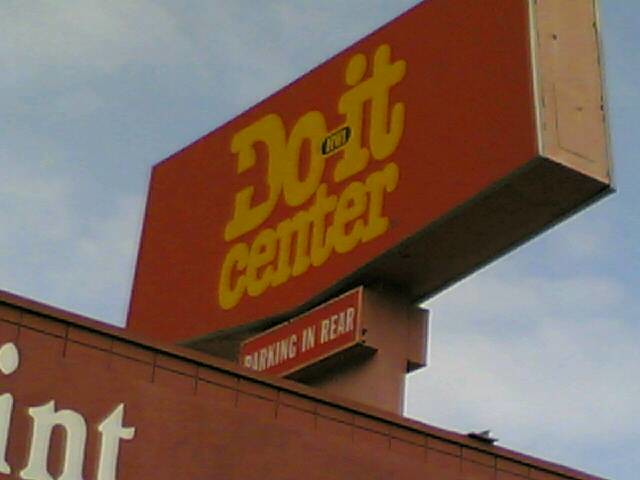This outdoor photograph, taken from a low angle during an overcast afternoon, features the top and roof of an industrial-looking building made of red concrete and brick. Atop the roof is a prominent rectangular sign with a weathered, rusty orange hue that reads "Do It Center" in bold yellow letters. Directly beneath it, there's a smaller red sign with white letters that says "Parking In Rear." The scene captures the simplicity of the sky with light, faint clouds against a muted, non-sunny blue background. Additionally, part of a white-lettered sign over an entranceway is visible, showing only the fragment "-INT" at the edge of the image. The focus is clearly on the signage crowning the building against the overcast, softly lit sky.